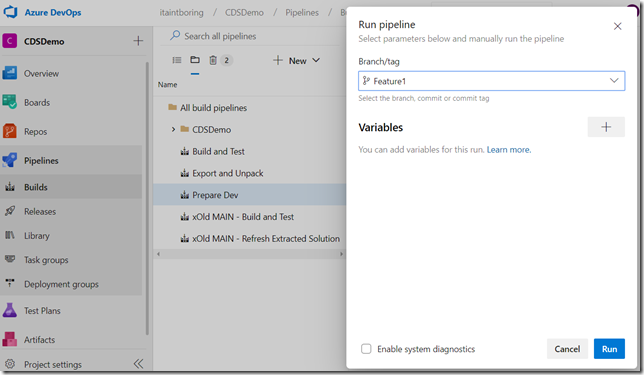A detailed caption for the image provided could be:

"This webpage is a screenshot from Azure D.E.V.O.P., a company specializing in development operations. The central focus is a square overlay positioned on the right-hand side against a white background. At the top of this overlay is the heading 'Run Pipeline' followed by smaller gray text indicating 'Select parameters below and manually run the pipeline.' Below, the overlay features a 'Branch/Tag' dropdown menu accompanied by a share icon showcasing 'feature one.' The directions 'Select a branch, commit or commit tag' are displayed beneath the dropdown. In bold black text, 'Variables' is labeled next, paired with a button containing a plus sign, suggesting users can add variables for the pipeline run. A blue link labeled 'Learn more' provides additional information. At the bottom of the overlay, a checkbox labeled 'Enable system diagnostics' is positioned next to two buttons: 'Cancel' and 'Run.' 

On the left-hand side of the image, a menu lists various options including CDS Demo, Boards, Repos, Pipelines, Builds, Releases, Elaborate, Test Groups, Deployment Groups, Test Plans, Artifacts, and Project One Settings. The background details are obscured by the square overlay, emphasizing the interactive elements of the pipeline configuration on the page."